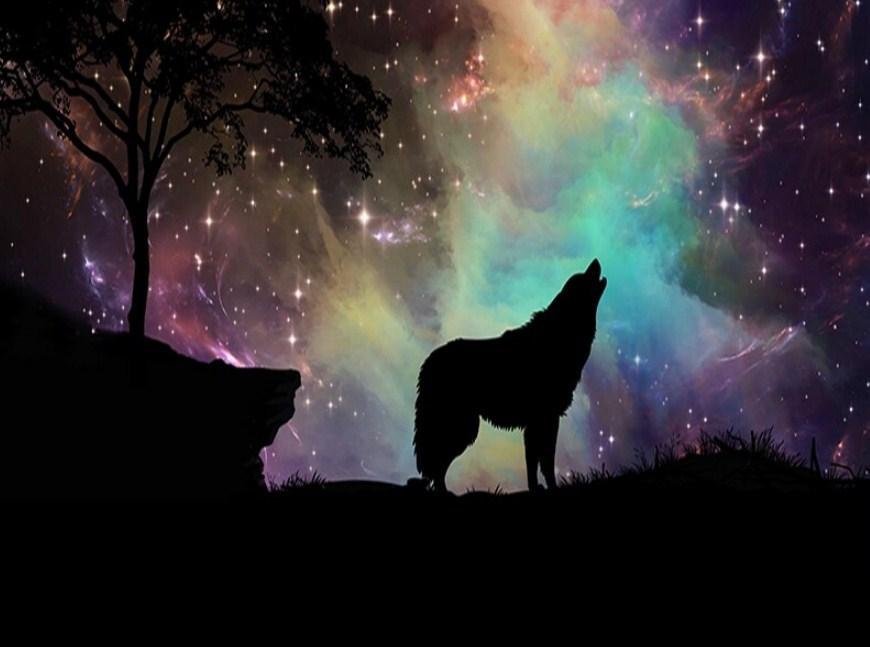The image depicts a black wolf, captured in a majestic and evocative scene, howling under a vibrant, starry night sky. The wolf, presented in silhouette, stands with its head lifted towards the heavens, mouth open in mid-howl, with its nose pointed skyward. This stance, along with its erect posture and downturned tail, indicates a powerful, almost mystical presence. The ground beneath the wolf is shrouded in darkness, possibly indicating it stands on a cliff or elevated surface, with a small tree visible on a higher portion to the left. The night sky is a breathtaking blend of turquoise, teal, yellow, purple, dark indigo, navy blue, and light blue hues, interspersed with sparkling white stars that give a sense of a magical, almost surreal atmosphere. This colorful backdrop contrasts beautifully with the wolf's dark silhouette, enhancing the overall drama and beauty of the scene.